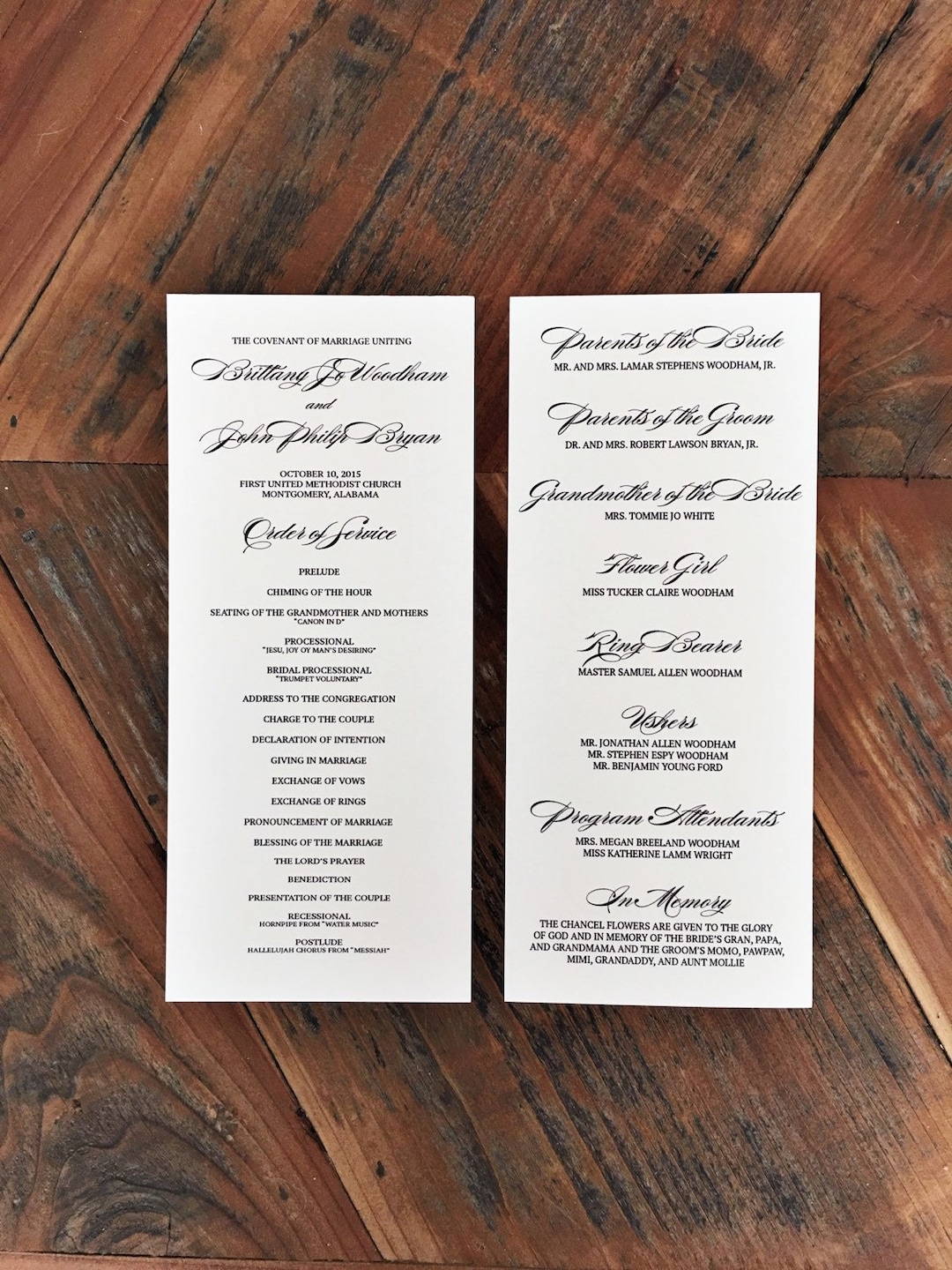This vertical rectangular image showcases an overhead view of two tall, white wedding program cards placed side by side on a dark wooden surface with visible planks and a distinctive grain pattern. Both cards have black text, with the one on the left detailing the "Covenant of Marriage" uniting Brittany and John on October 10th, 2015, along with the order of service for the wedding ceremony. The card on the right lists participants in the wedding, including the parents of the bride, parents of the groom, the grandmother, the flower girl, and the ring bearer, among others. The wooden surface has a rustic, deep brown hue that adds a charming contrast to the formality of the crisp, white cards.